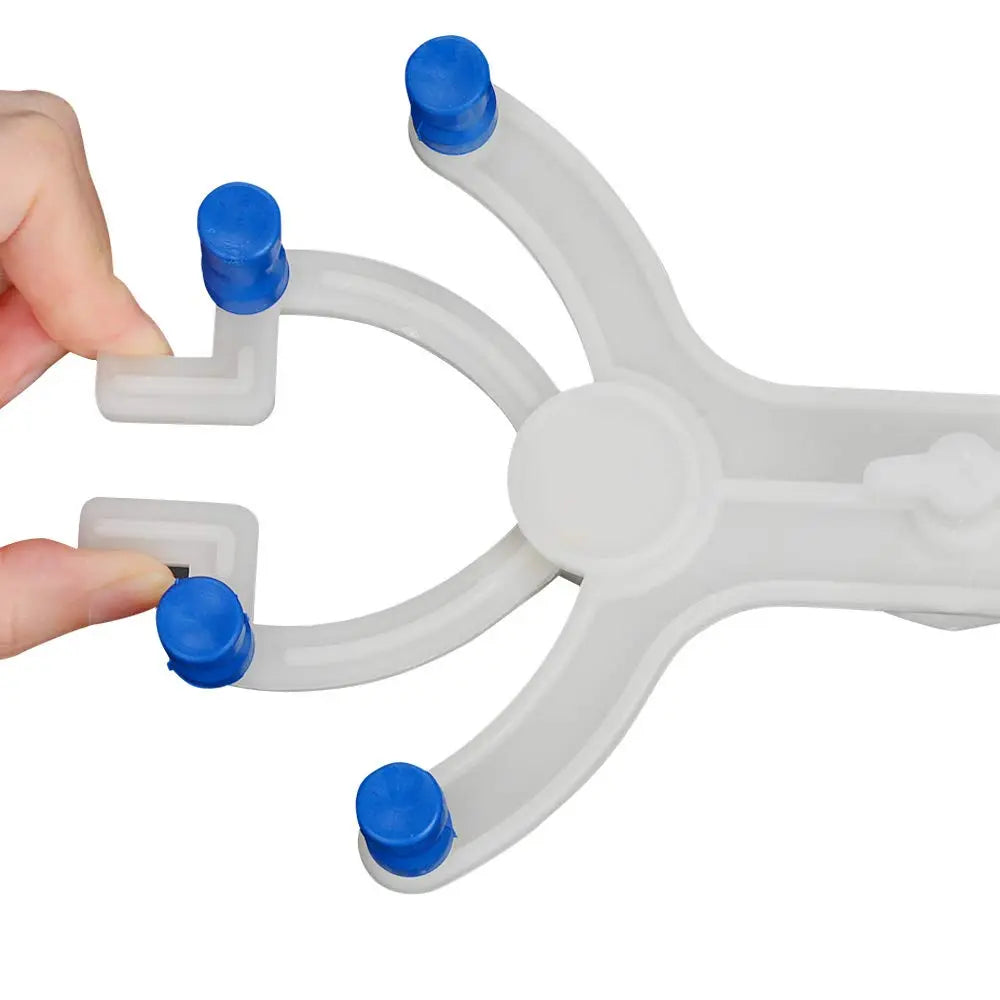In this image, set against a white background, a left human hand is prominently featured, grasping a peculiar grayish-silver plastic object. The object, resembling a Y shape with a V-shaped section in the middle, has a somewhat shield-like structure. The hand grips the upper ends of this 'shield' with the thumb and index finger, though the grasp does not seem to affect the apparatus. Notably, the object is adorned with four distinct blue knobs or caps, made from a rubber-like material, positioned at the ends of the Y and V shapes. These blue knobs stand out against the grayish body of the object, contributing to its unique and somewhat mysterious appearance.